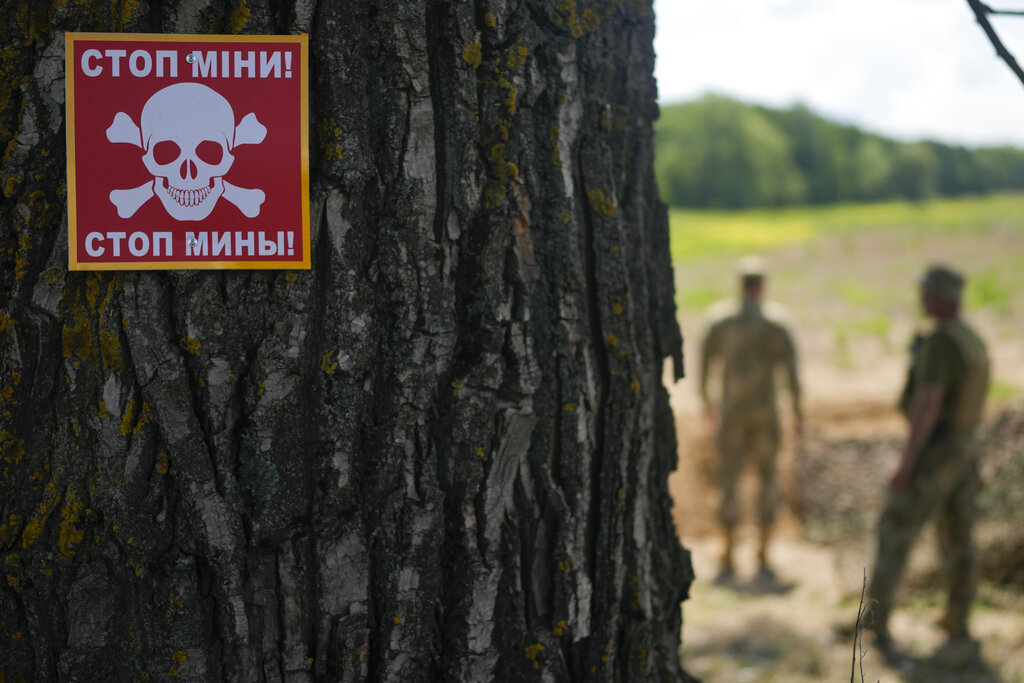The image depicts a close-up view of a tree trunk with a warning sign nailed to its bark in the foreground. The sign, which is square in shape and has a red background with a yellow border, features a white skull and crossbones, a universal symbol of danger. Written in white text, likely in Russian, the sign has characters that appear as "C-T-O-N M-I-H-N" with some letters seemingly reversed, followed by the phrase "C-T-O-N M-N-H-B-I!" Below and to the right of the tree, the blurred figures of two men dressed in military camouflage can be seen standing, seemingly gazing towards a large open field beyond them. The background reveals a vast expanse of green terrain with distant trees, suggesting the location might be an army range or a military site. The sharp focus on the tree and its warning sign contrasts with the softer, more blurred depiction of the soldiers and the distant field, emphasizing the danger indicated by the sign.